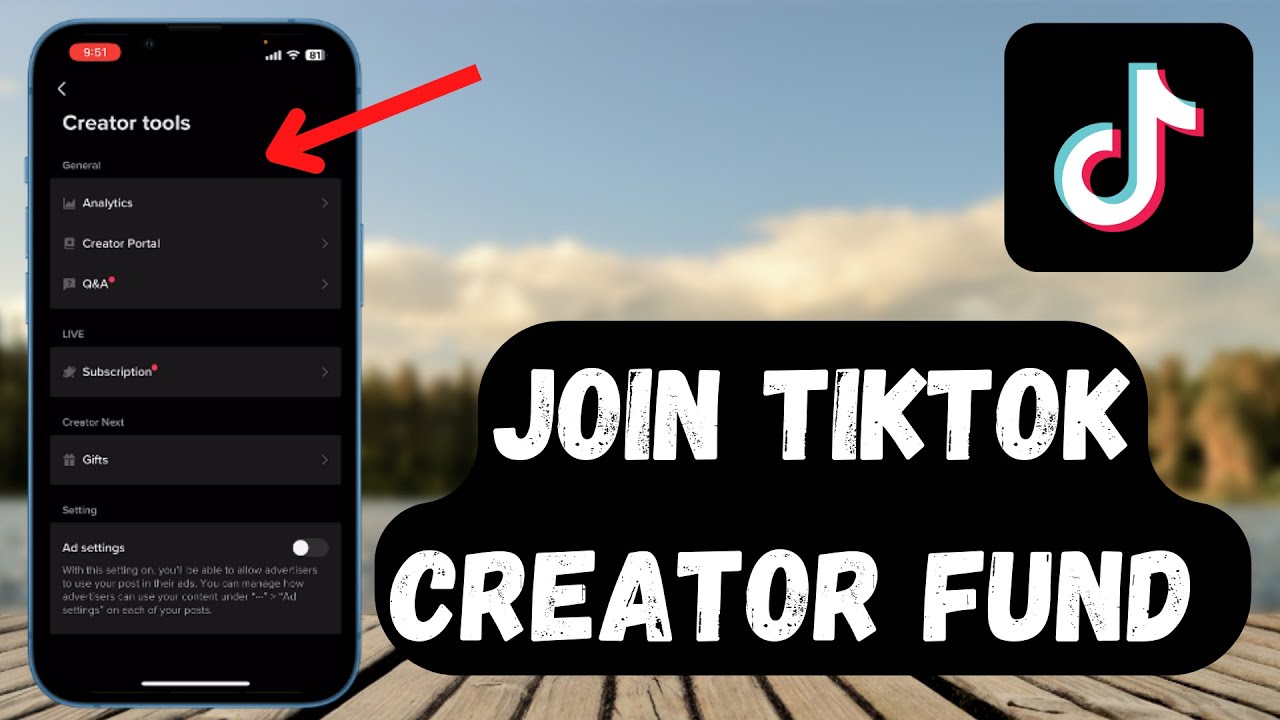In this visually engaging image, the top right features a black square showcasing the iconic TikTok logo, a sideways 'T' in white with a dynamic chromatic effect. The bottom middle of the image prominently displays a message encouraging participation in the TikTok Creator Fund, stylized with a black, paint-splotched background and white text that reads "Join TikTok Creator Fund."

On the far left, a smartphone is prominently featured, with a red arrow from the top middle left pointing towards it to draw attention. The phone's screen details are clearly visible: the top right shows a fully charged battery icon, a full Wi-Fi signal, and a full phone signal strength icon. The top left corner displays the time, which reads 9:51.

Beneath the time, the screen shows options listed under "Creator tools," starting with "General." Below this heading, three selectable categories are displayed: "Analytics," "Creator Portal," and "Q&A," the latter highlighted with a red asterisk, indicating importance or urgency. The overall composition directs focus to the features and tools available for TikTok creators, emphasizing the platform's support and resources.